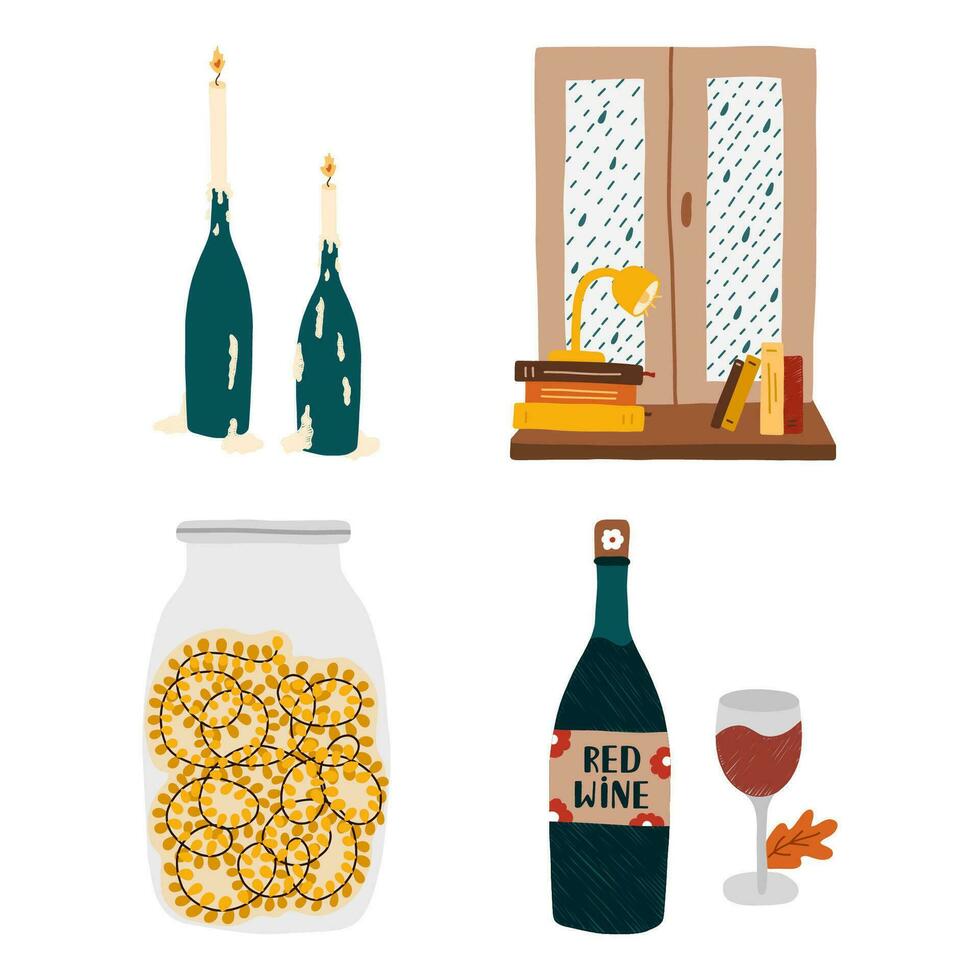The image depicts a collection of illustrated objects arranged in a cozy setting. At the top, there are white candles lit with flames, wax dripping down the sides, positioned in candle holders. To the right, a window is framed by a wooden shelf, adorned with a stack of books and a yellow desk lamp. Below this colorful tableau, on the bottom left, sits a glass jar filled with gold coins. Moving to the bottom right, a dark green bottle with a tan label reading "red wine" stands uncorked, accompanied by a full glass of red wine which appears to be swirling. An orange leaf delicately rests near the stem of the glass, adding a touch of autumnal charm to the scene.